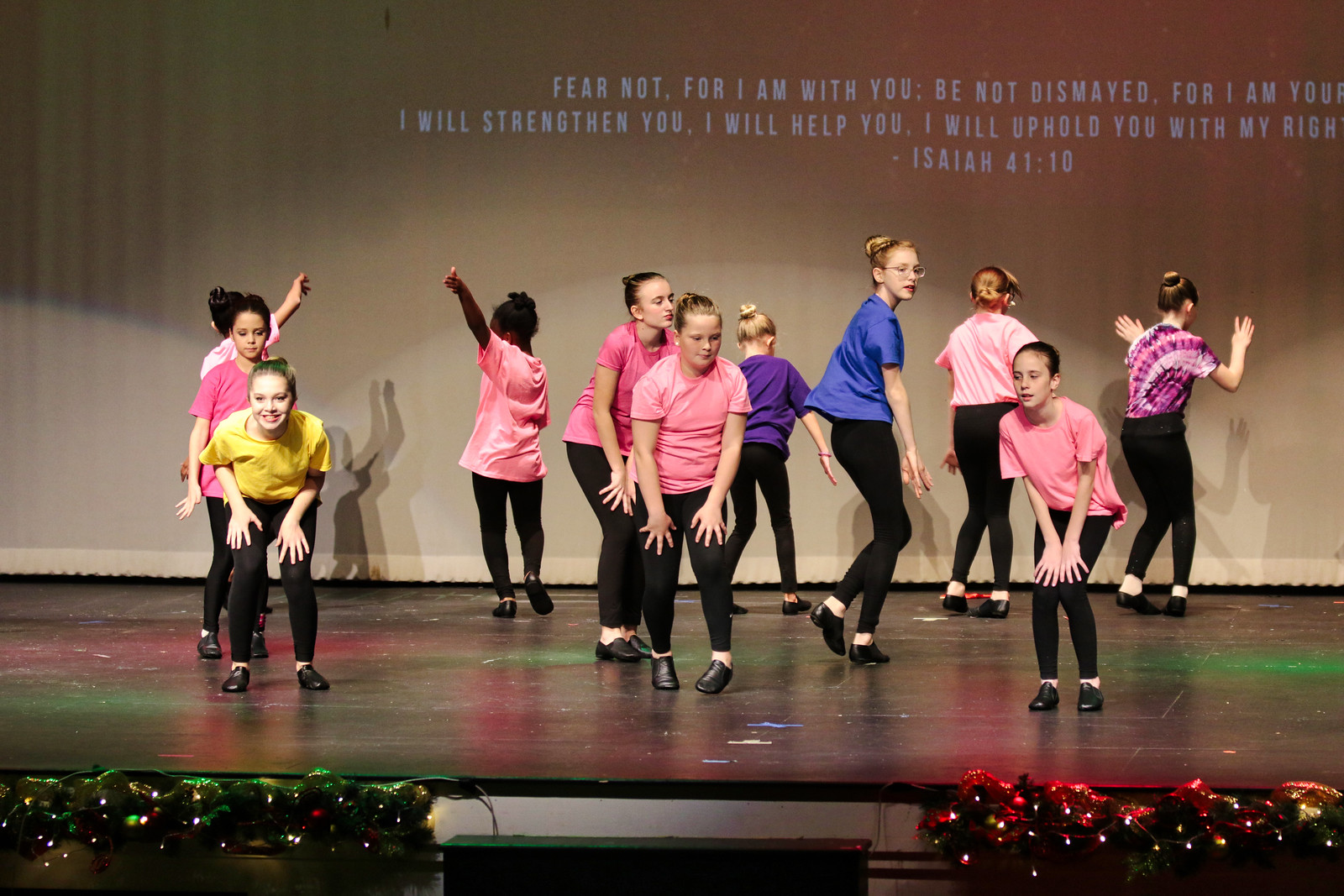The image depicts a lively dance performance featuring approximately 11 young girls on a wooden stage, with footlights casting a festive mix of green and red hues. The girls, likely pre-teens around 12 years old, are dressed in black pants and tap dance shoes, and are adorned in plain T-shirts of varying colors: pink dominates, but there are also noticeable yellow, purple, and blue shirts. The scene captures the participants in dynamic poses—some with hands on their knees and bent legs, others with arms raised, and a few with backs turned or standing sideways. Behind them, a projection on a brownish backdrop displays an inspirational quote, partly truncated: "Fear not, for I am with you. Be not dismayed, for I am your... I will strengthen you. I will help you. I will uphold you with my right... Isaiah 41:10." The performance exudes an energetic and perhaps festive vibe, reinforced by the stage lighting and the visible enthusiasm of the performers.